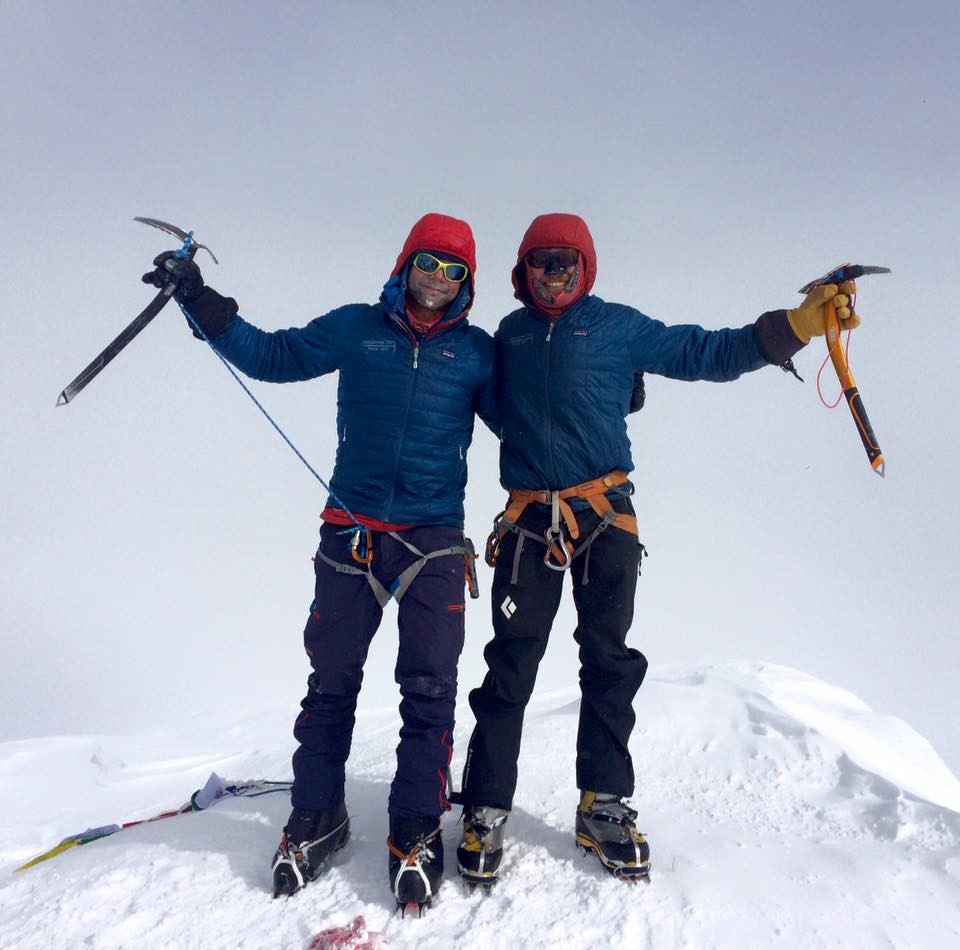In this detailed outdoor photograph, two tan-skinned male climbers stand arm in arm atop a snow-covered mountain summit, smiling with evident satisfaction. Both men are clad in matching blue jackets and red hoods, with harnesses and climbing equipment securely fastened around their waists. One climber wears navy blue pants while the other sports black pants, and they both have cleated climbing boots. Each climber holds a distinct pickaxe: the one on the left grips a black and silver pickaxe, while the one on the right holds a yellow and silver pickaxe. Completing their coordinated look, they each wear sunglasses—one with gold frames and the other with brown. The background is a pale whitish-gray sky, contributing to the chilling wintry atmosphere, with no other elements or people in sight, underscoring their impressive mountainous achievement.